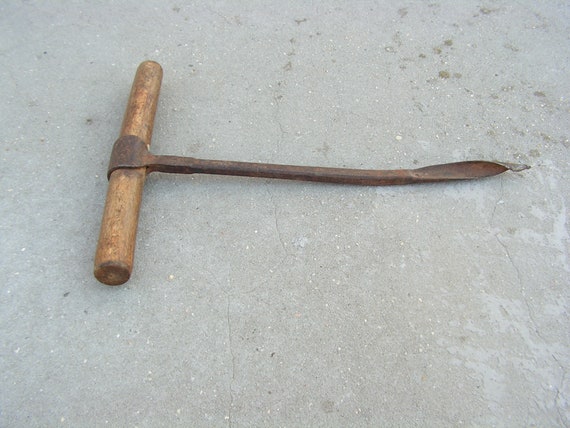The image showcases an aged and well-worn T-shaped hand tool resting on a gray cement surface, characterized by dark patches and some cracks. The horizontal part of the T, facing left, is a cylindrical wooden handle, light brown in color, visibly worn from extensive use. Attached to the center of this wooden handle is a long, rusty metal shaft, extending to the right, eventually tapering into a sharp, twisted point. The metal, darkened by rust, suggests significant age and use, and the overall design hints at a potentially multipurpose functionality, possibly for digging, scraping, or piercing. The worn condition of both the wood and metal emphasizes the tool's vintage and utilitarian nature.